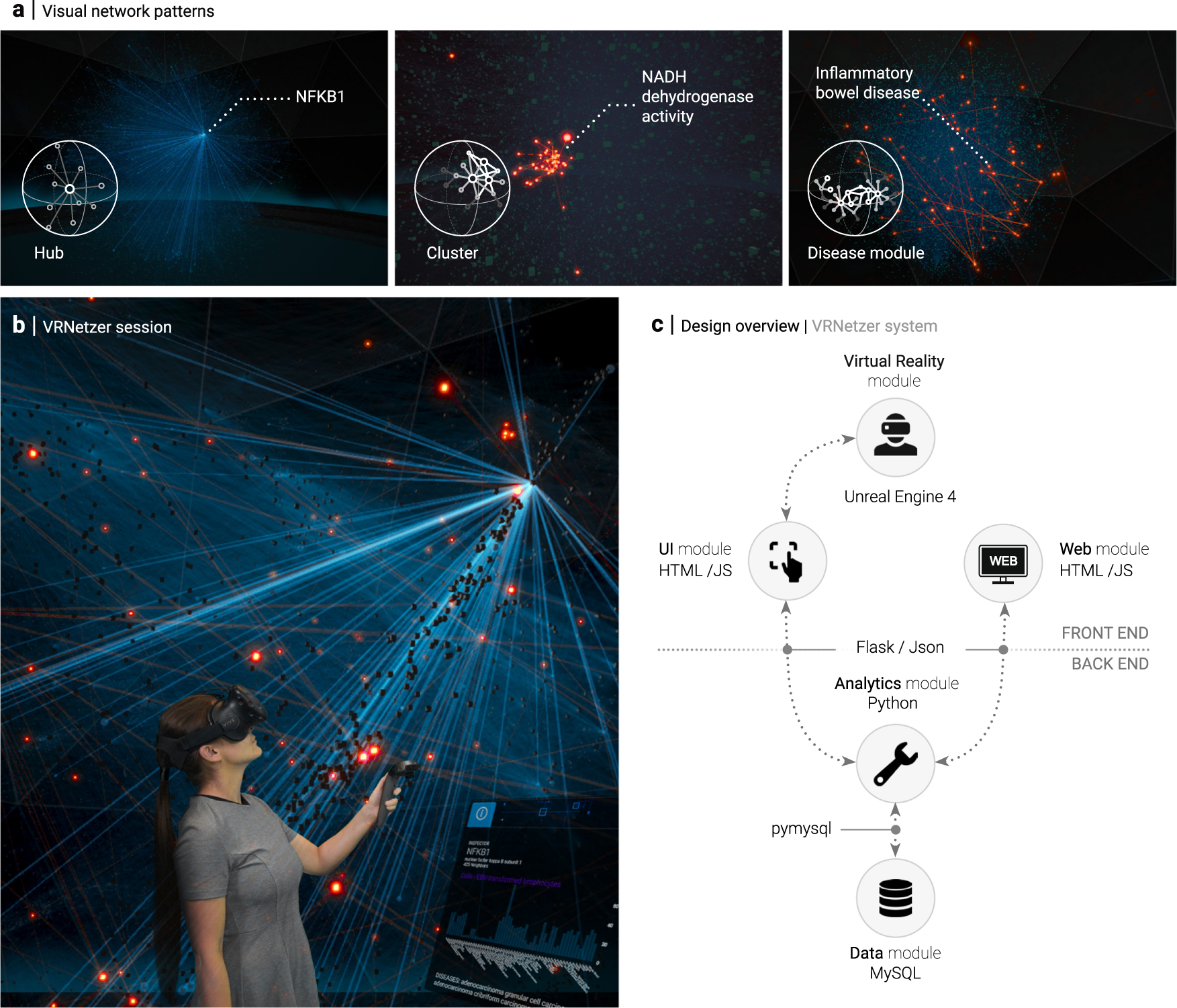The image is a detailed collage titled "Visual Network Patterns," consisting of five distinct sections. The top three images are representations of various scientific concepts connected to outer space-like constellations. Each section has a caption: the first on the left reads "hub" and features a blue light pattern with the label NFKB1. The middle image is labeled "cluster," depicting several red dots with the term NADH dehydrogenase activity. The rightmost image shows scattered red dots, captioned "disease module," and notes a link to inflammatory bowel disease.

Beneath these, the bottom left shows a woman in a gray shirt wearing a VR headset, holding a controller in her left hand. She is depicted interacting with a visual network of lights that includes clusters of blue and red dots projected around her. In the background, there's a monitor displaying various information.

The bottom right section is marked as the "design overview" for a virtual reality module, highlighting the use of Unreal Engine 4. It includes a comprehensive diagram detailing the VR system’s architecture, showing modules for user interface, data management, and analytics. The modules are associated with technologies like HTML/JavaScript, Python, Flask, JSON, and MySQL, differentiated between front-end and back-end components.